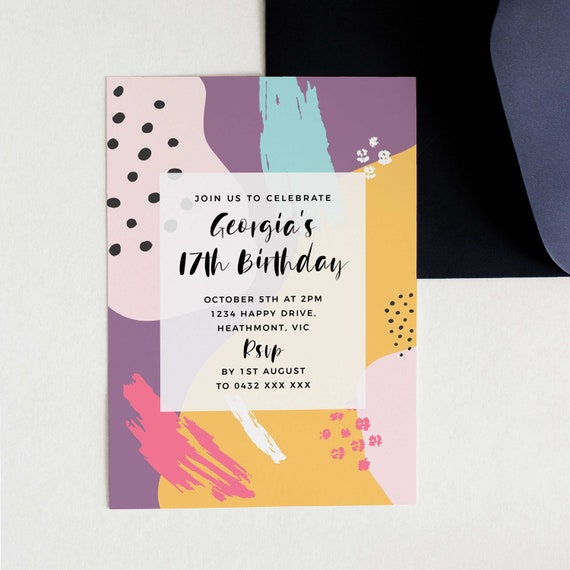The image is a detailed photograph of a birthday party invitation, positioned in the center against a white background. The upper right corner features a solid black envelope with its dark gray flap partially visible. The invitation itself is vibrant and colorful, exhibiting an abstract design with varied hues. Notably, there is a light pink blob with scattered black dots in the upper left corner, a pink brushstroke in the lower left that blends into a purple expanse reaching the upper right corner, and a yellowish-orange area in the lower left adorned with pink and black dots.

Centrally located on the invitation, a white square backdrop houses the textual details. At the top, in bold black typeface, it reads "Join us to celebrate," followed by "George's 17th Birthday" in a cursive font. Below, it specifies "October 5th at 2 p.m." and provides the address "1234 Happy Drive, Heathmont, Vic." The invitation also includes an RSVP note in cursive, requesting responses by "1st August 20432." The intricate blend of colors including light pink, purple, light blue, yellow, and white, along with the unique artistic elements, gives the invitation a festive and lively appearance appropriate for celebrating a 17th birthday.